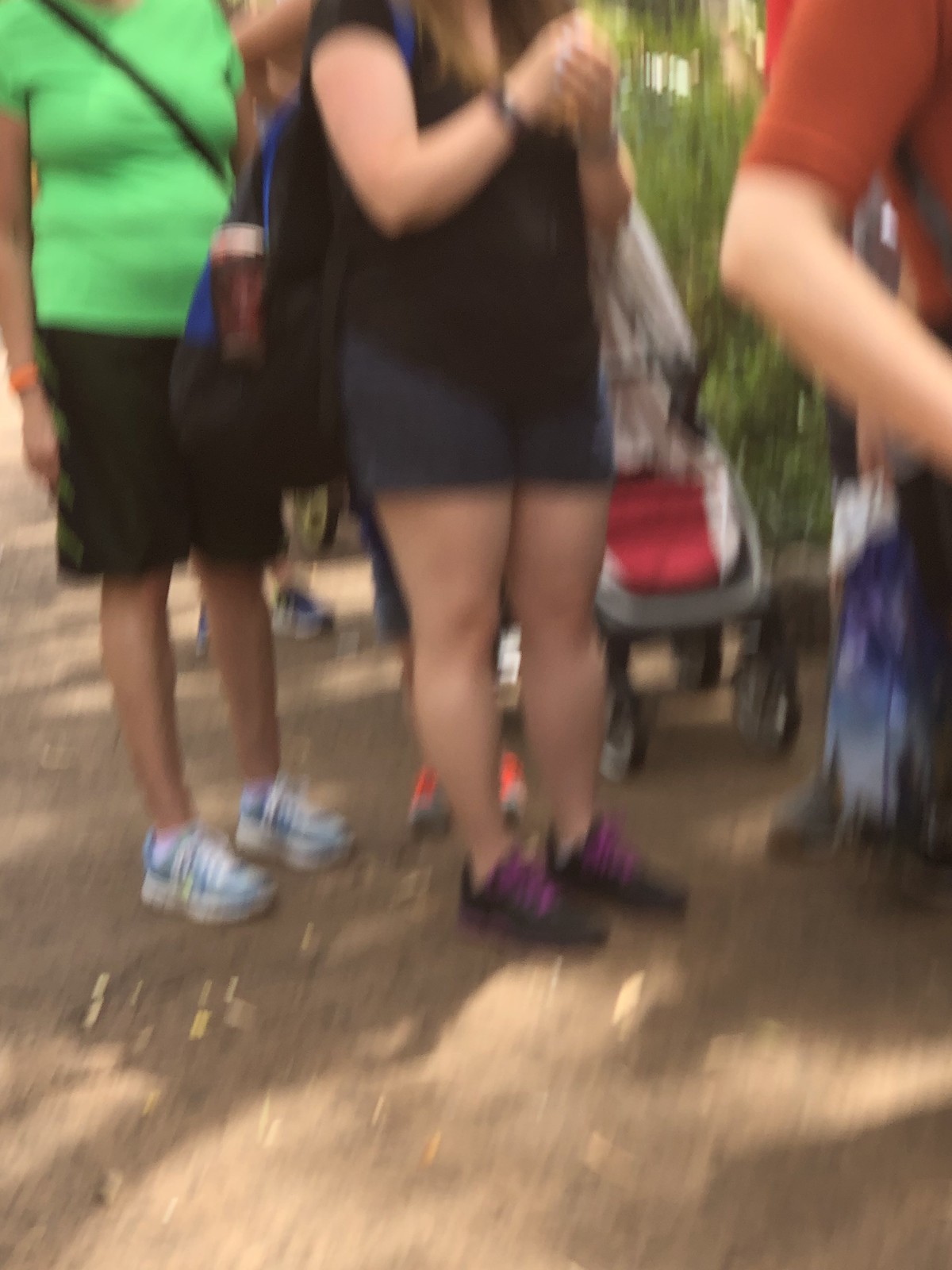A blurry photograph depicts several individuals standing in line, their bodies visible from the neck down. On the far left, a light-skinned woman is wearing a slightly tight green t-shirt, revealing a bit of her belly, paired with long black shorts. She sports white tennis shoes with blue edgings. In front of her stands a young, white-skinned woman dressed in dark blue jean shorts and a black t-shirt. She has a slightly fuller figure and wears black tennis shoes with purple shoelaces. This young lady carries a black bag that appears to hold a coffee cup, and a children's stroller is situated directly in front of her, from which the legs and shoes of a child can be seen. Additionally, an arm of a man in a rust-colored shirt is visible in front of her. The setting is outdoor, evident from the shadows cast on what seems to be a sidewalk, with a tree positioned behind the man.